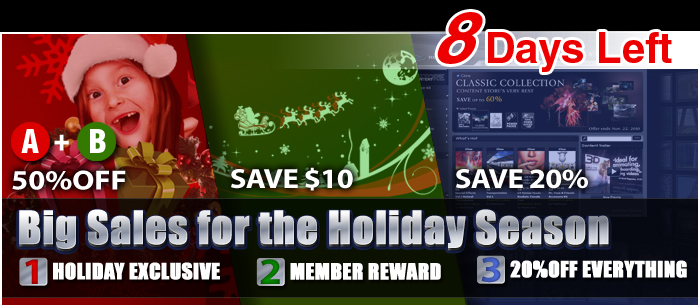In this vibrant Christmas-themed advertisement, the top section prominently features bold red letters against a white background, announcing "8 DAYS LEFT." On the left side of the image, a joyous little girl wearing a Santa hat beams widely, revealing a gap where her two front teeth are missing. Behind her, a festive red snowflake adds to the holiday spirit. Adjacent to her, a red circle with the letter 'A' and a green circle with the letter 'B' emphasize a promotional offer of "A + B = 50% OFF."

Further down, the background transitions to green, depicting Santa Claus in his sleigh pulled by reindeer with a text overlay proclaiming "SAVE $10." Below this, a bluish section features the phrase "CLASSIC COLLECTIONS," accompanied by assorted festive images and a discount offer of "SAVE 20%."

The bottom portion of the ad highlights "BIG SALES FOR THE HOLIDAY SEASON," outlining several exclusive offers: "1. Holiday Exclusive, 2. Member Reward, 3. 20% Off Everything." The overall composition is filled with vivid colors and cheerful holiday imagery, enticing viewers with incredible festive savings.